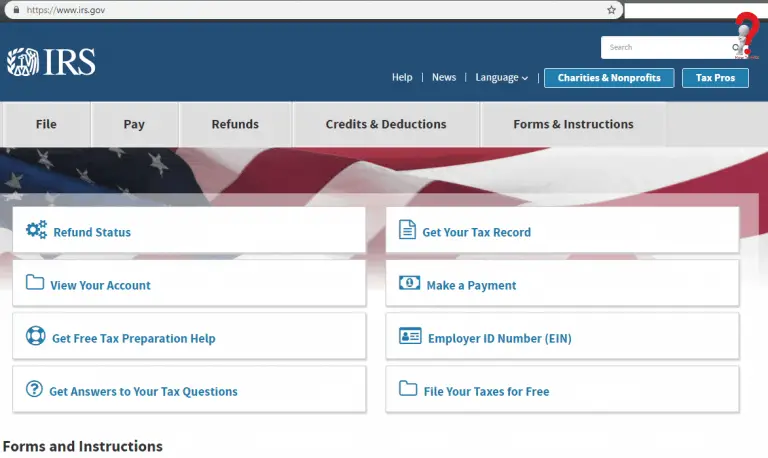Screen capture from the official IRS homepage located at www.IRS.gov. The page features a blue header containing the IRS logo and a search bar. Highlighted navigation options include "File," "Pay," "Refunds," "Credits and Deductions," and "Forms and Instructions." Additionally, a red question mark, which is not native to the page, is visually present indicating user-added emphasis. Below the main categories, various resources are listed: "Refund Status," "View Your Account," "Get Free Tax Preparation Help," "Get Answers to Your Tax Questions," "Get Your Tax Record," "Make a Payment," and "Employer ID Number (EIN)," along with "File Your Taxes for Free." Further navigation options, such as "Help," "News," "Language," "Charities and Nonprofits," and "Tax Pros," appear under the main tabs. The screenshot also includes an image of an American flag, enhancing the government-related theme.